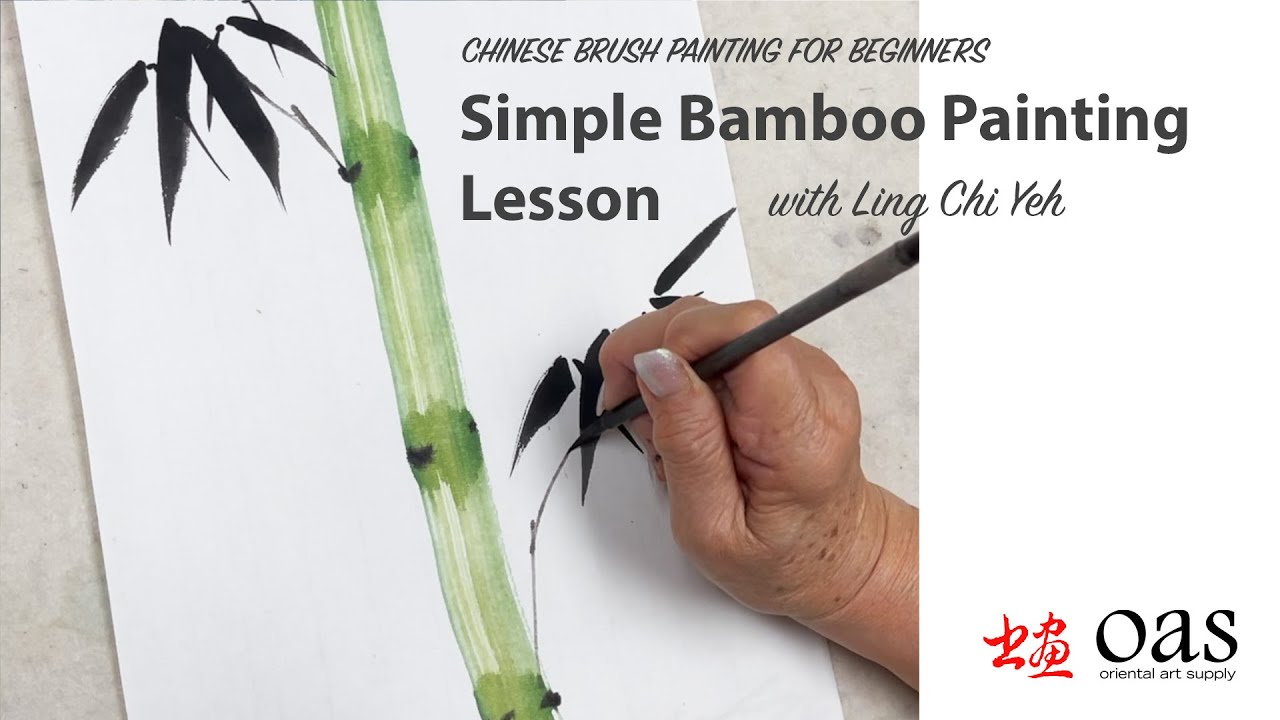The image is a computer-edited advertisement for a beginner's Chinese brush painting lesson with Ling Jie. It prominently features the slightly aged and sun-spotted hand of an older individual, with long, shimmery-polished fingernails, delicately painting a bamboo stalk and leaves on a white piece of paper using a thin black paintbrush. The bamboo is depicted with vibrant green hues and dark leaves. In the upper portion of the image, there is text that reads, "Chinese Brush Painting for Beginners, Simple Bamboo Painting Lesson with Ling Jie." On the right side of the painted bamboo, there is a red Chinese symbol followed by the initials "OAS" in black, and below it, in smaller font, the words "Oriental Art Supply." The advertisement appears to be set against a stone-like table surface with clear details that highlight its instructional purpose and artistic theme.